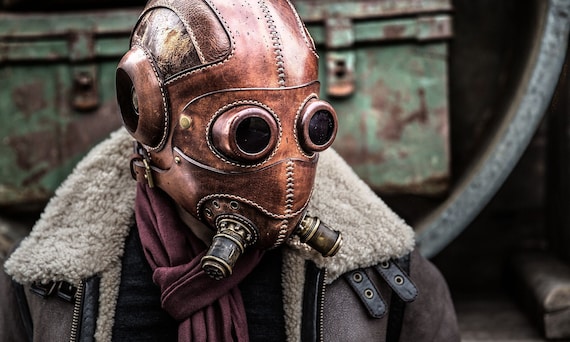In this detailed photograph, a humanoid figure is adorned with a steampunk-inspired gas mask known as the "Dust Angel," a skull helmet crafted from various layers of industrial leather in shades of golden gray and brown with a glossy finish. The full-head covering mask features small round integrated eyepieces made of copper, cylindrical breathing apparatuses resembling brass canisters with drilled holes at the mouth area, and elaborate ear coverings with metal dome-shaped openings. A strap with a buckle is situated just below the left ear. Over the mask, the individual wears a dark black bomber jacket, characterized by its white Sherpa fleece collar. The jacket is open, revealing dark purple clothing underneath and a red scarf. The background accentuates the industrial theme, with blurred metal surfaces, including walls and chests equipped with clips, clasps, and hoses lending an atmosphere reminiscent of a Star Wars setting.